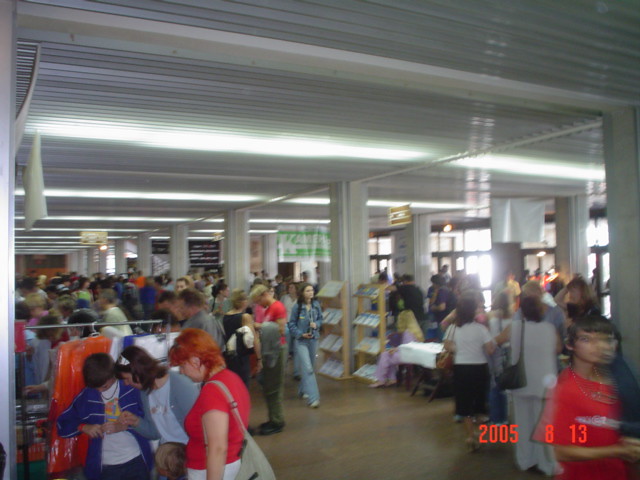The photograph captures a slightly out-of-focus, rectangular indoor scene of a bustling vendor market or craft sale set in a large room. The room features tall white pillars that divide the space and provide structural support. The brown wooden floor is visible at the bottom of the image, enhancing the warm ambiance of the space. Fluorescent lights embedded in white ceiling panels illuminate the entire area, casting a bright, even light over the scene.

In the lower left-hand corner, a group of three people is engaged, seemingly focused on the items displayed. A clothes rack draped with clothes wrapped in plastic occupies this section, hinting at the variety of goods available. Towards the middle left-hand side, a larger crowd mills about, moving from one display to the next, contributing to the dynamic atmosphere of the market.

Tables set up with various items, along with shelves holding books or brochures, are interspersed throughout the room. On the right-hand side of the image, an entire wall of windows floods the space with natural sunlight, enhancing visibility and adding to the overall warmth of the environment. Red numerals "2005, 8, 13" are noticeable in the lower right-hand corner, possibly marking a date.

Overall, the photo captures a vibrant, bustling indoor market scene with numerous people engaged in browsing and shopping amidst an array of household goods and clothing.